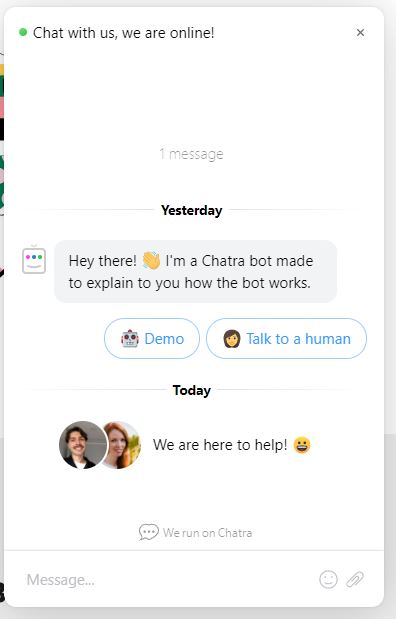A smartphone screen displays an open chat interface on a white background. At the top right corner, there is a tiny box with an "X" for closing the chat. To the top left, the text "Chat with us, we are online!" is prominently displayed next to a green dot indicating online status. Below these elements is some blank white space, followed by the message "1 message" in gray.

A thin gray line bisects the screen horizontally, with "Yesterday" in bold black letters centered on this line, indicating the following messages are from the previous day. The chat includes an icon of a classic robot with a gray outline, a little antenna on top, three eyes in red, blue, and green, and a gray smiley face. The chat bot's message is on a gray background and reads, "Hey there! 👋 I'm a chat robot made to explain to you how the bot works. I'm Chatra."

Below this text, there are two interactive options with blue outlines and text. The left option says "Demo" accompanied by a robot emoji 🤖, and the right option says "Talk to a human" with an emoji of a woman with brown hair 👩.

Further down, a caption "Today" in black marks the start of messages sent today. There are two profile photos: a young man with dark hair and a mustache, overlapping a young woman with long red hair. Their combined message reads, "We are here to help! 😀" with a smiling emoji. Below this, there is a speech bubble with three dots, indicating someone is typing, and the text "We run on Chatra." There's a text entry box labeled "Message..." alongside icons for a smiley face and a paper clip, likely for sending emojis and attachments.